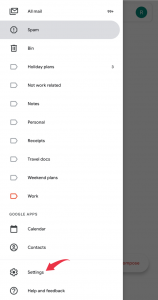The image appears to be a screenshot of a drop-down menu from a computer or phone screen. On the left side of the screenshot, there is a prominent white bar, and to the right of that white bar is a gray area. The gray area seems to be part of someone's email interface. At the very top of the interface, there is a section labeled "All Mail," though it is blurred out and somewhat difficult to read. Directly below this top section is a gray bar. 

Continuing downwards, the interface displays several lines of text on a white background with black lettering. Near the bottom of the screenshot, there is an entry second from the bottom featuring a gear icon on the left side. To the right of the gear icon are the words "Settings." Additionally, there is a red arrow drawn to the right of the word "Settings," pointing directly at it for emphasis. 

In the upper right corner of the image, within the gray area, there is some more text that appears to be in the background, along with a noticeable circle. The entire screenshot gives the impression of navigating through the email settings menu.